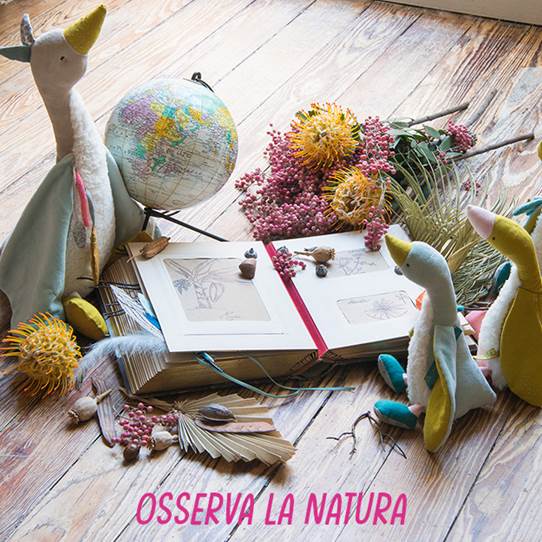This image shows a charming scene set against a brown wooden floor with a sliver of a beige wall in the background. Three stuffed ducks are prominently featured: the leftmost, resembling a mother goose with a white coat and a yellow bill, and two baby ducks to the right, one with blue feet and the other with a pink bill. Surrounding them is an assortment of whimsical objects. A colorful globe sits beside the mother goose, adorned with lines of latitude and longitude and elevated on a stand. An open book with a red spine, featuring hand-drawn illustrations, lies in front of the baby ducks. Scattered around are dried flowers in various hues of yellow, pink, green, and brown, alongside some fallen leaves. At the very bottom of the image, the words "Observa la Natura" appear in pink, capitalized text. This endearing setup seems designed to evoke a theme of nature and learning, blending soft toys with educational and natural elements.